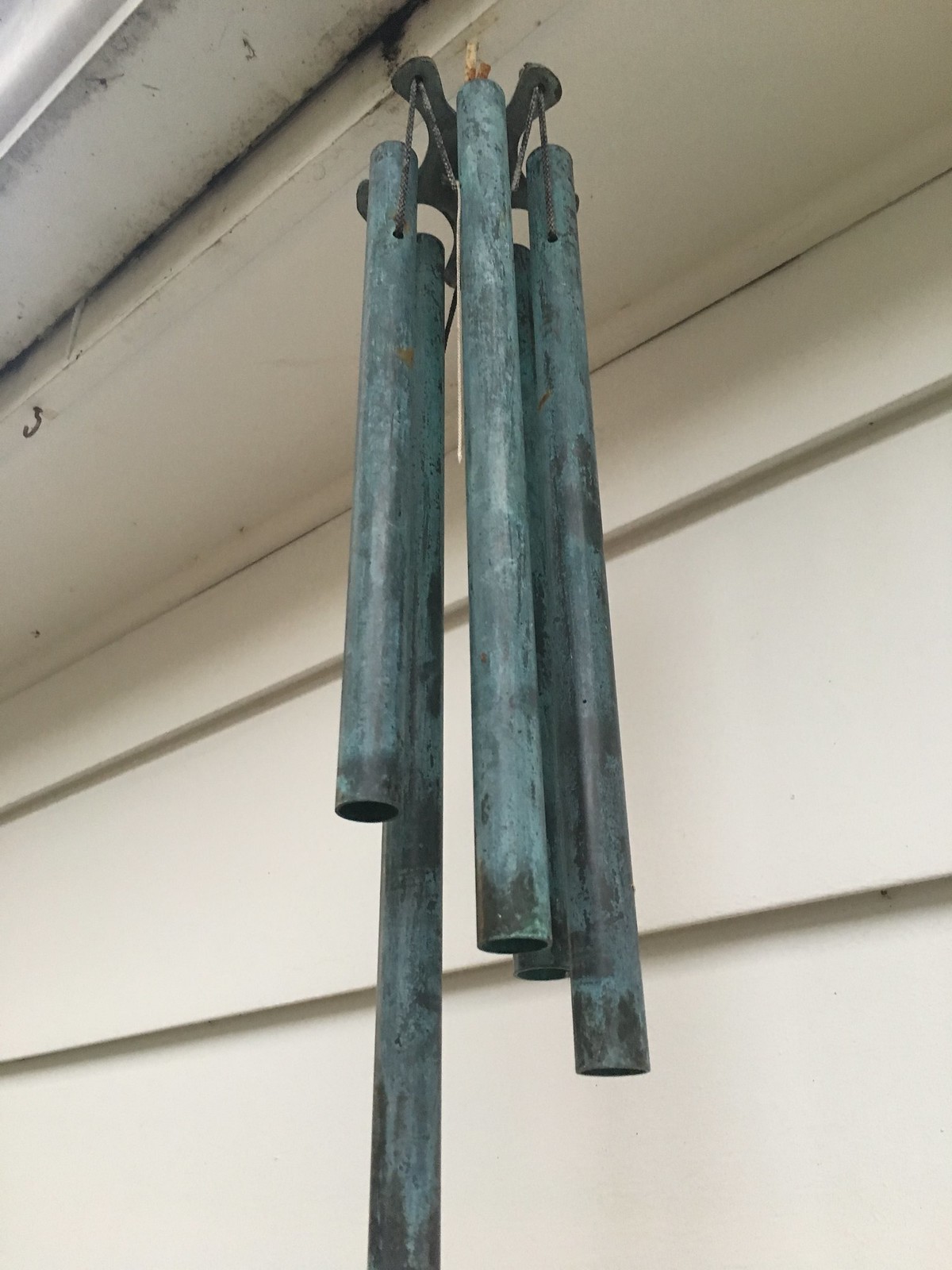This photo showcases a set of tarnished, greenish metal wind chimes hanging from the underside of an eave beneath a gutter. The chimes consist of five metal tubes, each of varying lengths, with the longest tube positioned at the back. These tubes are connected by strings to a star-shaped metal ring. The wind chimes, which catch the wind and produce a melodic, bell-like noise, are suspended from a hook embedded in a white-painted board at the top of the roof. The structure behind the chimes has white vinyl siding. The siding and wooden parts of the house appear slightly dirty and stained, featuring another nearly invisible hook used to secure the wind chimes.